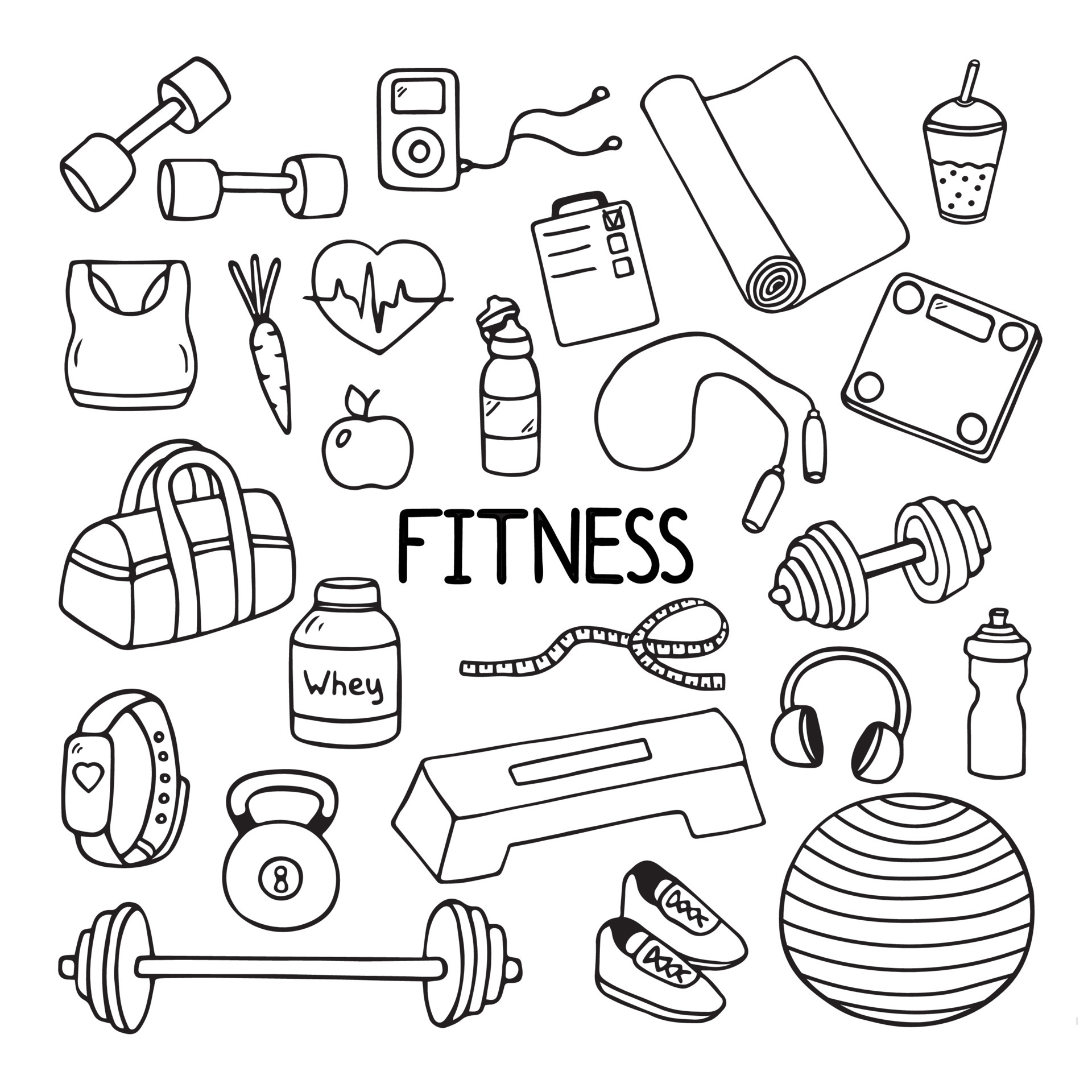The illustration revolves around the central theme of "FITNESS," prominently displayed in black capital letters. Encircling the central word is an assortment of meticulously drawn items that represent various aspects of fitness and health. To the left, there are hand weights (dumbbells), and adjacent to them is an MP3 player accompanied by headphones, suggesting motivational music for workouts. 

Nearby sits a yoga mat, ideal for stretching and flexibility exercises. Below the mat is a shaker bottle with a straw, hinting at hydration and nutrition on-the-go. A high-tech scale capable of measuring body composition, including body fat and water content, is also illustrated.

On the right side, a jump rope hints at cardio exercises, while a large barbell and a separate kettlebell represent strength training. Over-the-ear headphones indicate immersive workout sound. A Pilates ball is included, signifying core and balance training, alongside another shaker bottle tailored for hydration.

A step platform used for aerobic step exercises, a pair of athletic shoes, and a free-weight barbell further emphasize varied workout routines. An illustrated smart watch hints at heart rate monitoring with a tiny heart icon, while a jar labeled "WEIGH" suggests a nutritional supplement. 

The collection is completed with a measuring tape for tracking physical changes, another water bottle with a pop-off lid, a fresh apple, and a heart rate line symbol synonymous with health monitoring. Also featured are a crunchy carrot, a supportive sports bra, and a practical gym bag, encapsulating the comprehensive essentials for anyone dedicated to fitness.